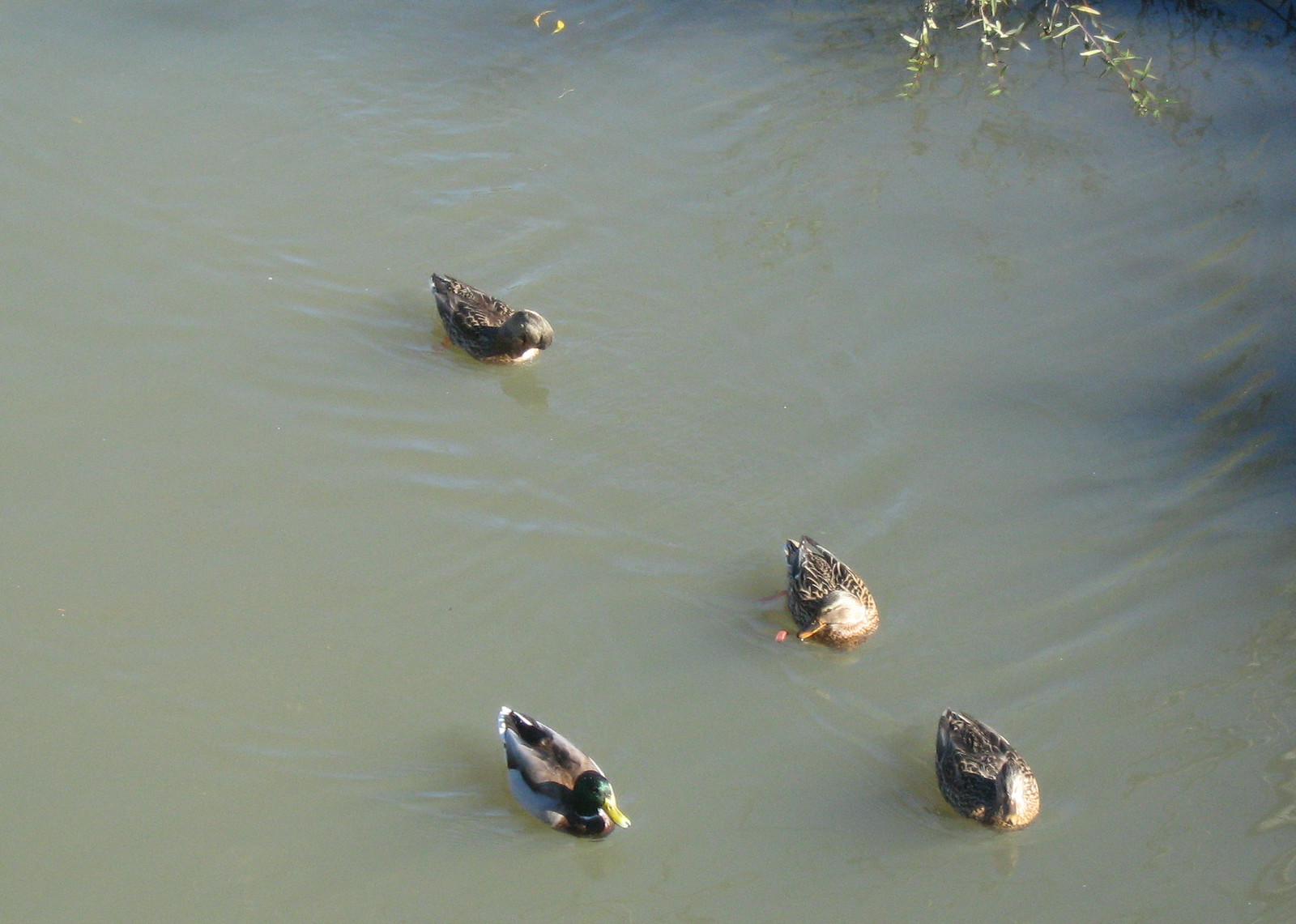In this photograph, four ducks are swimming in murky, brownish-green water, which appears nearly opaque. The majority of the frame is filled with this water, showing ripples trailing behind the ducks as they swim forward. Among the ducks, there is one male mallard distinguished by his vibrant green head and yellow bill, positioned on the left side of the image. The remaining three ducks appear to be females, featuring more subdued grey and white plumage with pale to orange bills. These three ducks are aligned in a row, swimming towards the bottom right of the frame. One of the female ducks has its head turned sideways, possibly peering at something small and brown in the water, while another has its head submerged, feeding. In the background, a few branches of a tree or bush hang down into the pond, adding a delicate detail to the scene dominated by water and waterfowl.